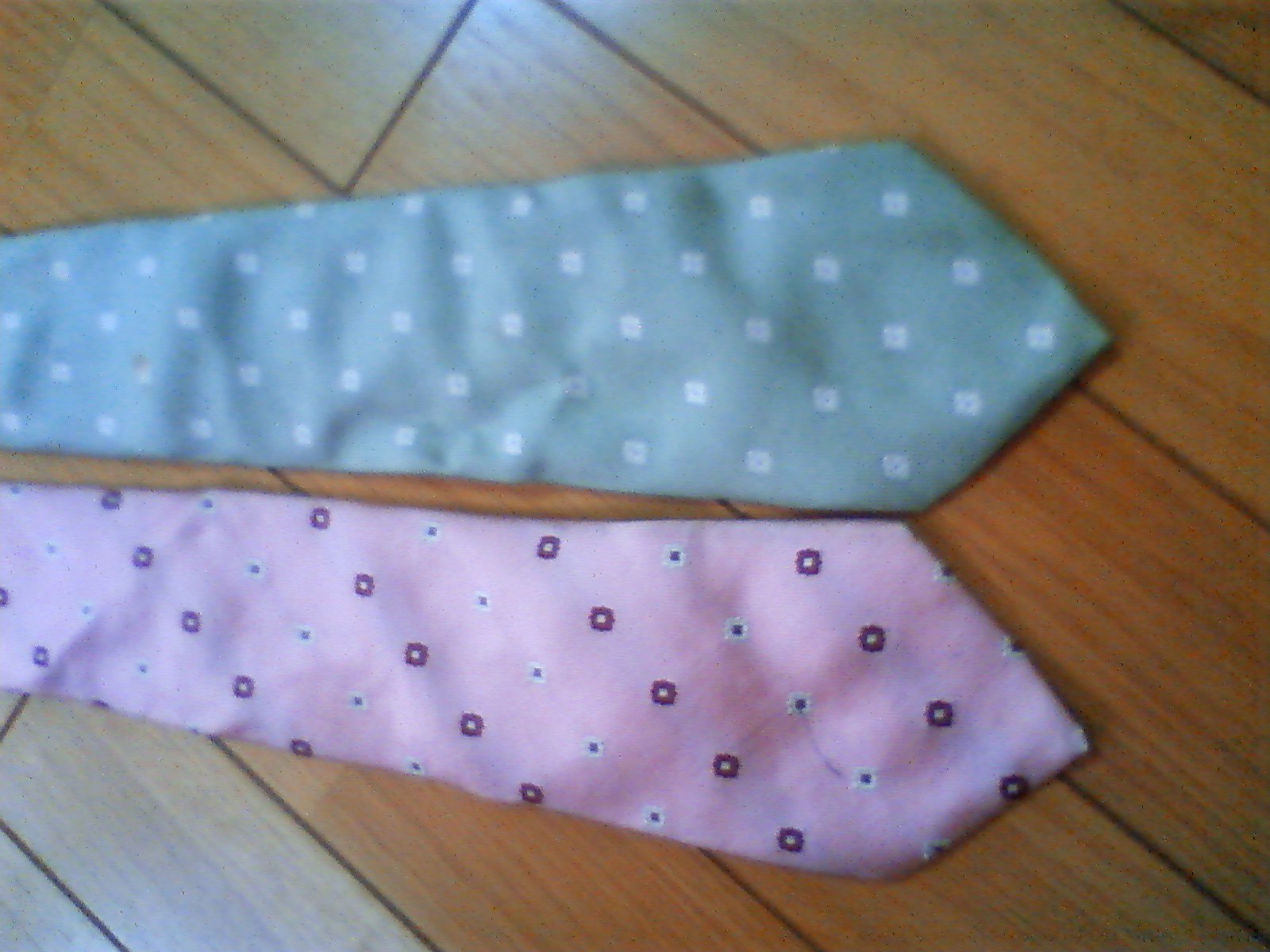The photograph captures two neckties laid out on a light-colored wooden surface, likely a hardwood floor or a wooden table, featuring distinct planks of wood joint together. The ties are positioned with their V-shaped ends facing right. The tie on top presents a pale turquoise shade adorned with a diagonal pattern of white shapes that align into lines whether observed from the left or right. The lower tie displays a pink base interspersed with symmetrical patterns of lavender and white circles, some featuring pink or black dots at their centers. Only the lower halves of the ties are visible, showcasing their average width.